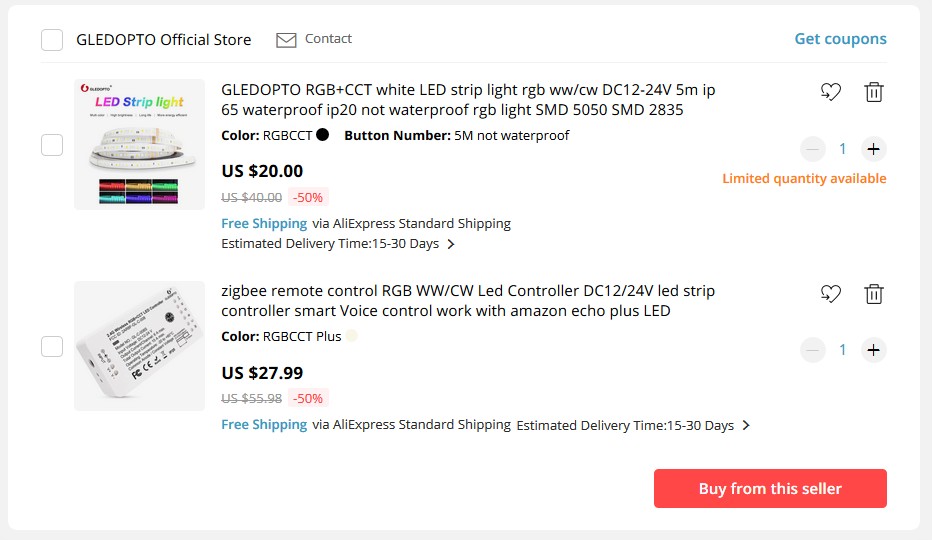In the image, two separate products are being listed on a sales page from the GLEDOPTO Official Store. 

At the top left, a square logo is displayed beside the store name "GLEDOPTO Official Store." To the right of this, there's an email icon labeled "Contact." The top right corner features a blue button that says "Get Coupons."

The first product listed is the "GLEDOTPORGBCCTYLEDSTRIP65WPIP20NWPRGBLIGHTSMD5050SMD2835." Accompanying this product name is an image of LED strip lights, showcased with vibrant rainbow text that reads "LED Strip Light." The LED strip lights are priced at USD $20, marked down from their original price of $40, reflecting a 50% discount. This discounted price is highlighted in red text. The product offers free shipping via AliExpress Standard Shipping, with an estimated delivery time of 15 to 30 days. Further down, orange text announces the limited quantity available. The quantity selected is 1.

Below this listing, the second product is a "Zigbee Remote Control RGB." This controller is compatible with Amazon Echo Plus. Priced at $27.99, it originally cost $55.98, also showing a 50% discount. The product also features free shipping through AliExpress Standard Shipping. The selected quantity for this item is 1, displayed in blue text.

At the bottom right corner, a white text within a red rectangle prompts users to "Buy from the seller."